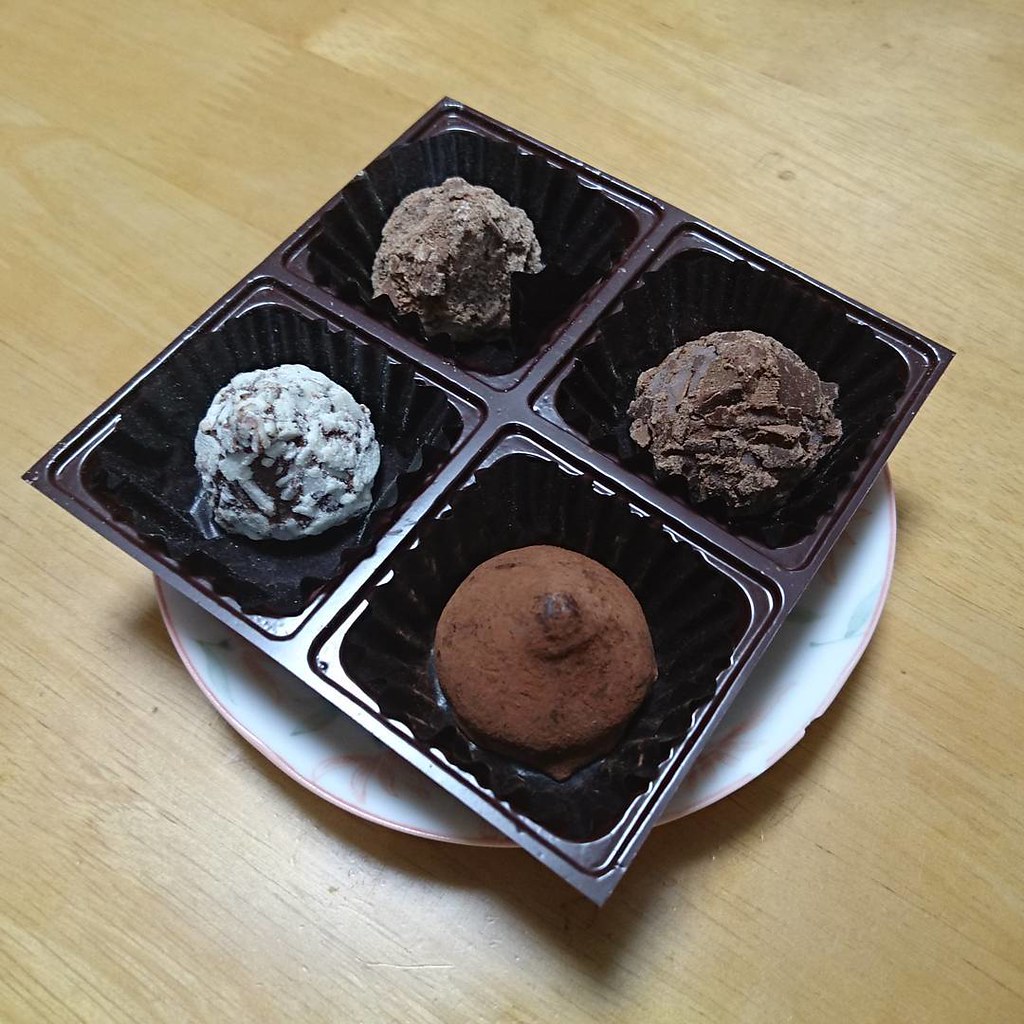In this detailed image, a light golden-colored wooden tabletop prominently features a white china plate with a distinctive pink and blue ring along its chipped edges. Centrally positioned on the plate rests a black plastic container divided into four compartments, each hosting a unique piece of chocolate dessert that resembles truffles or chunky chocolate cupcakes. The compartment at the top contains a smooth brown chocolate piece, while the one on the right holds another brown chunk that appears slightly rougher. To the left, there's a chocolate piece with a grayish-green hue, and the bottom section houses a light brown chocolate chunk with a dusting that could be powdered sugar. This focused composition includes no other objects or text, allowing full attention to the elaborately detailed desserts and their elegant yet simple presentation.